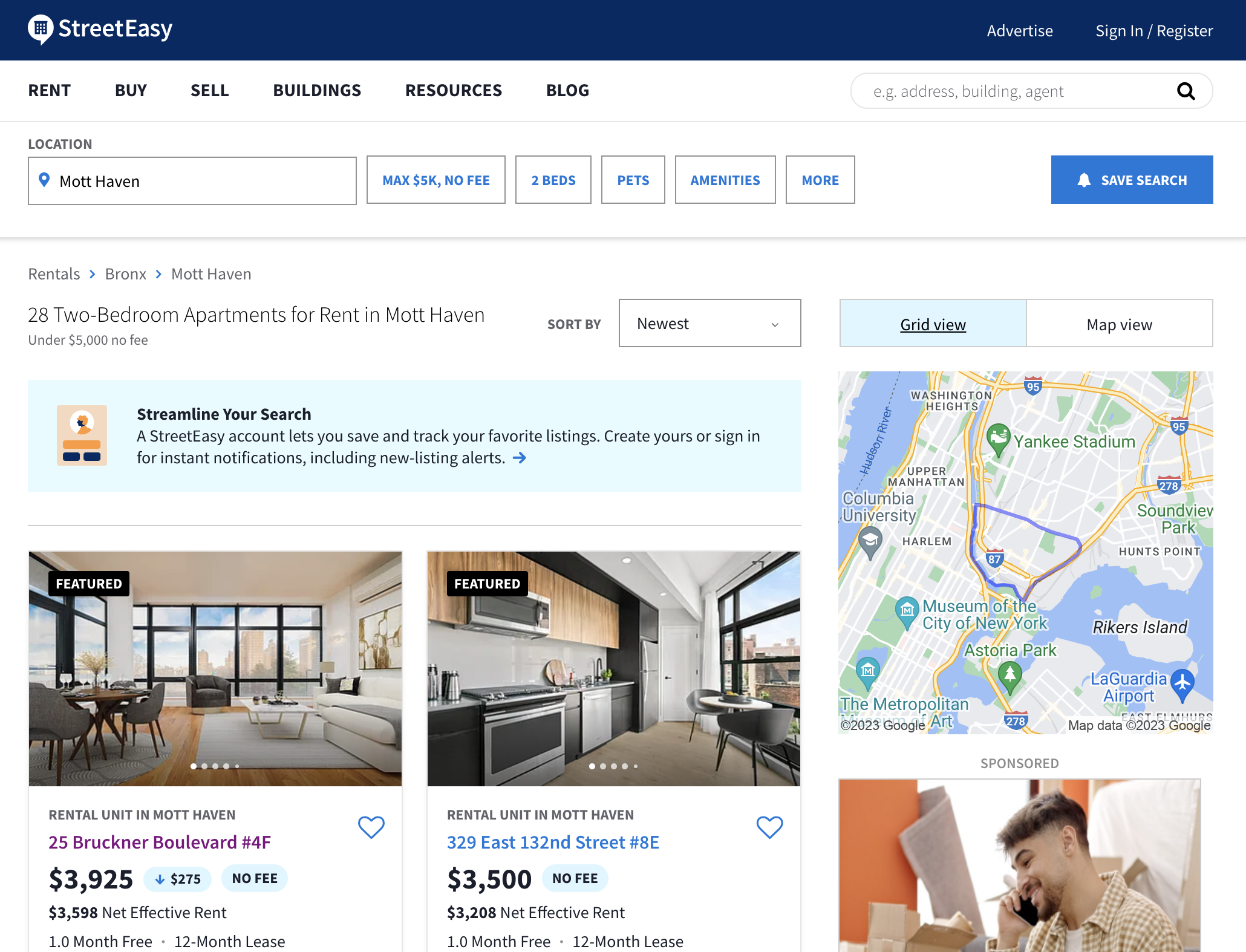A screen capture of the StreetEasy website showcasing various apartment listings in Mott Haven. The top of the site features a blue navigation bar with the StreetEasy logo, along with options to "Advertise," "Sign In," and "Register." Below, there is a secondary navigation menu with categories such as "Rent," "Buy," "Sell," "Buildings," "Resources," and "Blog." The central search box displays current filters: location set to "Mott Haven," a maximum price of "$500,000," and criteria including "no fee," "two beds," "pets," and "amenities." A blue "Save Search" button is also visible next to these filters.

Directly beneath the search bar, the display indicates that there are "28 two-bedroom apartments for rent in Mott Haven, under $5,000," with a sorting option set to "newest." The listings start with a "Featured" label, showing a photo of a rental apartment. The first listing highlights a rental unit at 25 Bruckner Boulevard, Apartment 4F, priced at $3,925. Adjacent to it, another image showcases an apartment located at 329 East 132nd Street, Apartment 8, listed for $3,500.